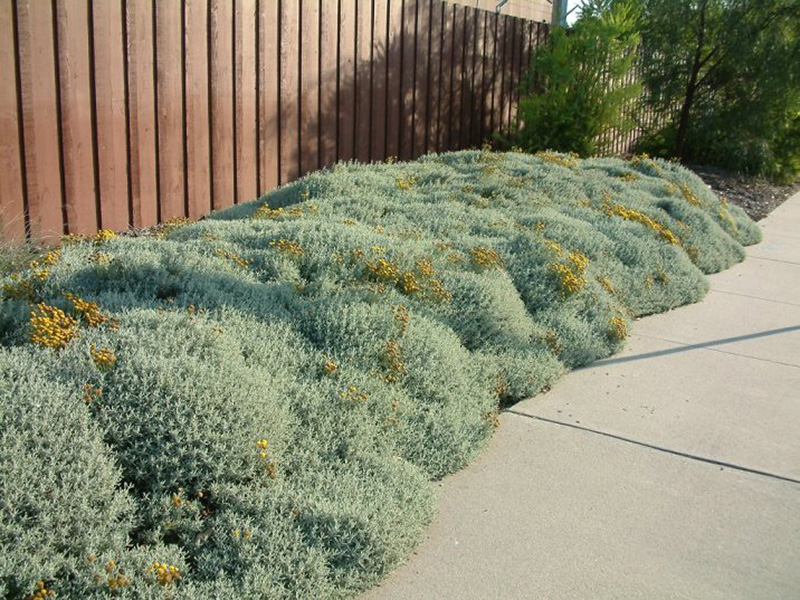This landscape-oriented image captures a suburban scene featuring a sidewalk in the lower-right corner. Parallel to the sidewalk, a well-maintained wooden picket fence with vertical dark wood slats stretches from the left side of the image to the center. Alongside the fence, dense ground cover of bushy, light bluish-green (almost turquoise) plants with clusters of yellowish-golden flowers adds vibrant color. This landscaped area also features patches of dark brown wood chips. In the background, partially obscured by the fence, the upper portion of a house peeks out, along with a sliver of the sky visible behind a tall, full tree. This tree, along with a few other trees, provides canopy and greenery on the right side of the image and casts shadows over the scene, adding depth and contrast. The overall setting is a neatly landscaped, serene outdoor walkway area with a mix of natural and man-made elements.